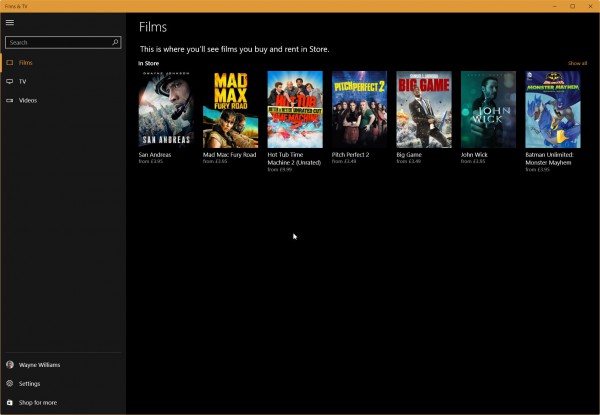The image is a detailed snapshot of a website that appears to be similar to IMDb, showcasing a selection of films available for purchase and rental. The main section displays seven movie titles: "San Andreas," "Mad Max: Fury Road," "Hot Tub Time Machine 2 (Unrated)," "Pitch Perfect 2," "Big Game," "John Wick," and "Batman Unlimited: Monster Mayhem." At the top right of this list, a yellow text button labeled "Show All" invites users to explore more titles.

On the left-hand side of the screen, a hamburger menu provides navigation options including "Search," "Films," "TV," and "Videos." Below this, the user profile of Wayne Williams is displayed with a small circular icon beside it. Further down, gear and store icons are present, labeled "Settings" and "Shop for More," respectively. 

The upper right corner features a yellow banner with the text "TV & Films," emphasizing the range of content. Standard window control buttons for minimizing and closing the window are present here as well. The background of the website is black, with white text providing clear contrast.

The film images are vibrant, presenting a mix of colors such as yellow, blue, pink, red, and dark gray, adding visual interest to the black and white interface.